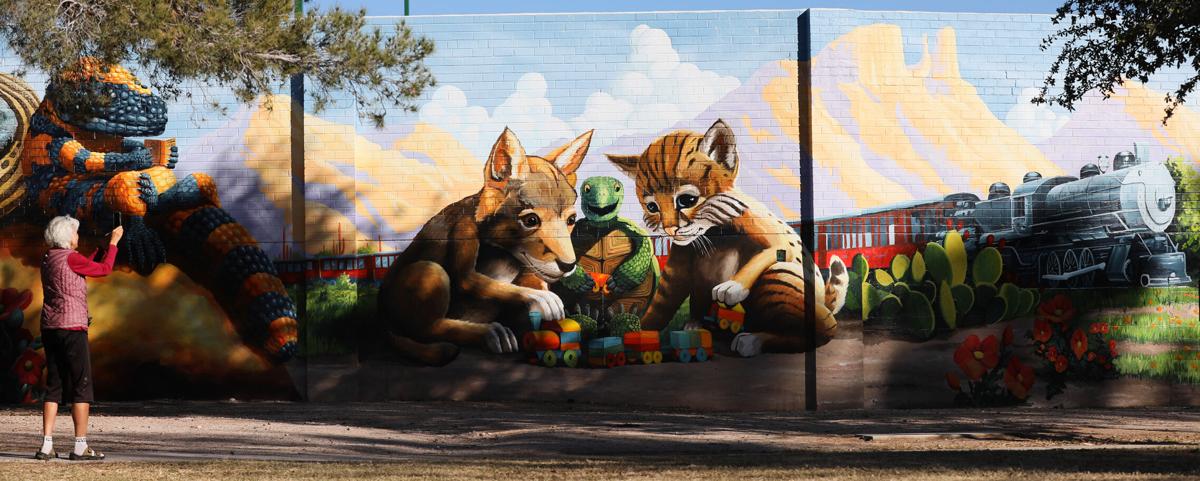This image is a highly detailed mural painted on the side of a building, capturing a whimsical scene of a fox and a cat playing with blocks, while a green turtle looks on from between them. The fox, positioned on the left, is brown, and the cat on the right is a dark brown-orange with white and black stripes on its face. An elderly woman in the foreground, wearing a purple jacket with red sleeves and black pants, is photographing the mural. She is also wearing socks with sandals. Above her, a striking blue and orange lizard-like creature is perched. The mural spans three sections of the wall; the left section features large leaf plants and a gray amphibian with orange stripes, while the right section depicts a silver locomotive train with a red car arriving at a station, which connects visually with the middle section through the cat's tail extending into this scene. The background shows a blue sky with clouds and hints of yellow sunlight, adding a lively atmosphere to the mural.